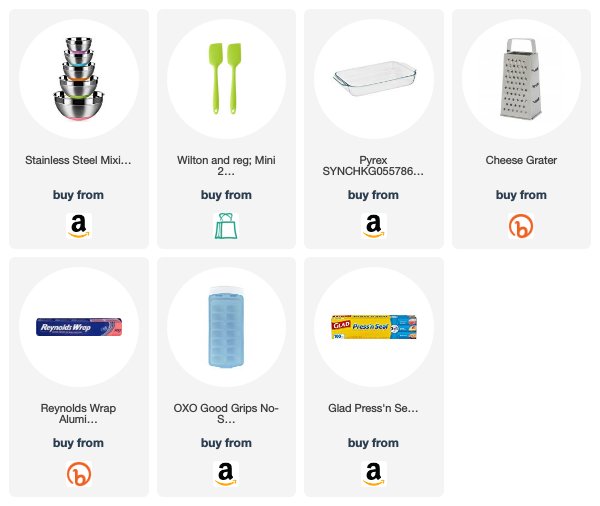The image features a grid of seven gray boxes arranged in two rows, with four boxes on the top row and three boxes on the bottom row. Each gray box includes a small white oval shape near the top, which seems to be for labeling purposes. 

The contents of the boxes are as follows:

1. The top left box displays a metal object labeled "Stainless Steel Mixing ..." with a call-to-action to "Buy from Amazon."
2. The top middle-left box showcases two green spatulas labeled "Wilton and Wray Mini 2 ..." accompanied by a grocery bag icon for the purchase option.
3. The top middle-right box contains a clear baking pan with the label "Pyrex Sink KG 055786," and it also prompts the user to "Buy from Amazon."
4. The top right box features a metal cheese grater labeled "cheese grater," with a circular icon containing the letter 'B' indicating the purchasing option.
5. The bottom left box is unspecified in the provided text.
6. The bottom middle box is unspecified in the provided text.
7. The bottom right box displays a yellow cardboard box labeled "Glad Press and Seal," with a "Buy from Amazon" option.

The various items range from kitchen utensils to storage solutions, each with clear instructions on how to purchase them from different platforms.